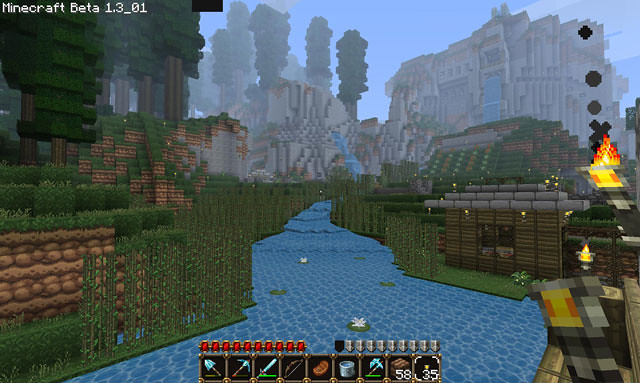The image appears to be a screenshot from the Minecraft Beta 1.3-01 game. The scene features a tall castle-like structure against a bright blue sky. Surrounding the castle are large trees and various grey buildings highlighted with brown lines, adding texture and detail. A striking blue waterfall cascades alongside these buildings, adding a scenic element.

On the right side of the image, there's a prominent, primarily grey building with splashes of blue and other colors. The bottom of this structure features grass-covered steps. Towards the right, vibrant yellow and red flames are visible, accompanied by small dots, possibly representing embers or sparks. Below the flames, there seems to be a fortress-like construction made of brown materials, complete with pipes on the top and a wall with mixed green and brown hues on the left side.

The floor is predominantly blue with a lighter blue maze-like design interwoven across it. At the bottom of the image, a series of red dots are visible alongside boxes containing various items such as axes. Additionally, there are more boxes on the right side of the screen with small silver icons above them, which are likely indicators or buttons that may light up during gameplay.